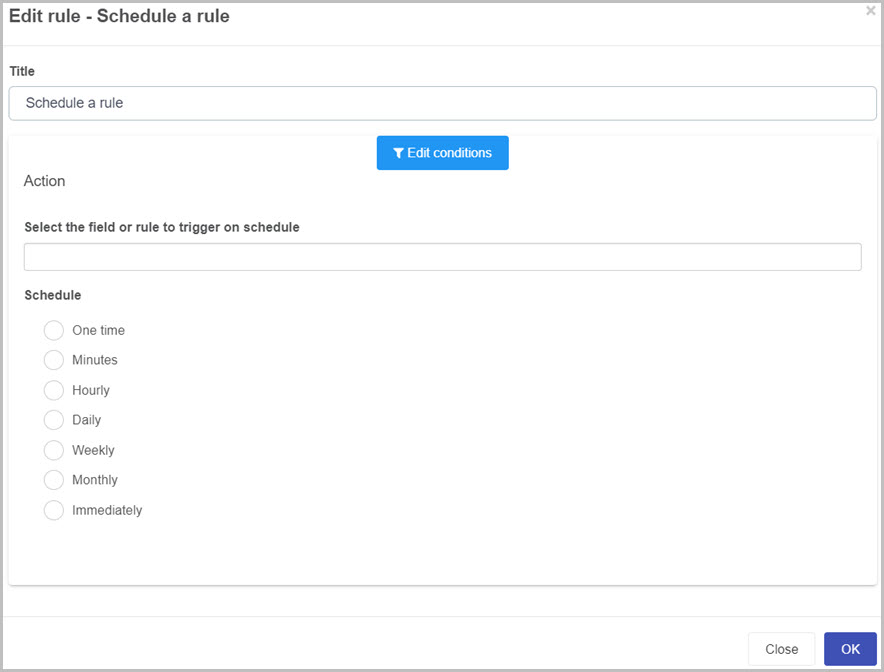This is a detailed screenshot of a homepage with a minimalistic white background, encased by a dark gray border. In the top left corner, the text "Edit Rule - Schedule a Rule" is prominently displayed in bold black font. On the top right side, there is a small gray "X" icon. 

Beneath the header, a thin gray line stretches across the width of the page. Just below this line, aligned to the left, the word "Title" is bolded in black. Directly under it, there is a long rectangular input field spanning the entire width, containing the placeholder text "Schedule a Rule."

In the center, beneath the input field, a blue button labeled "Edit Conditions" is visible. Moving back to the left side, under the "Action" heading (similarly styled in bold black), there is smaller, semi-bolded black text instructing users to "Select the field or rule to trigger on schedule." Below this instruction is another long rectangular input field.

Continuing downward, the text "Schedule" is bolded in black. Directly below the letters "E" and "D," there are several white circles with light gray borders, each one representing a scheduling option. From top to bottom, these circles are accompanied by labels: "One Time," "Minutes," "Hourly," "Daily," "Weekly," "Monthly," and "Immediately," all in-line with the corresponding circle on their left.

At approximately one inch below this section, a horizontal gray line extends across the page. In the bottom right corner, there is a blue button featuring the word "Okay" in white text. To its left, a smaller white button with a thin gray border is labeled "Close" in gray text.